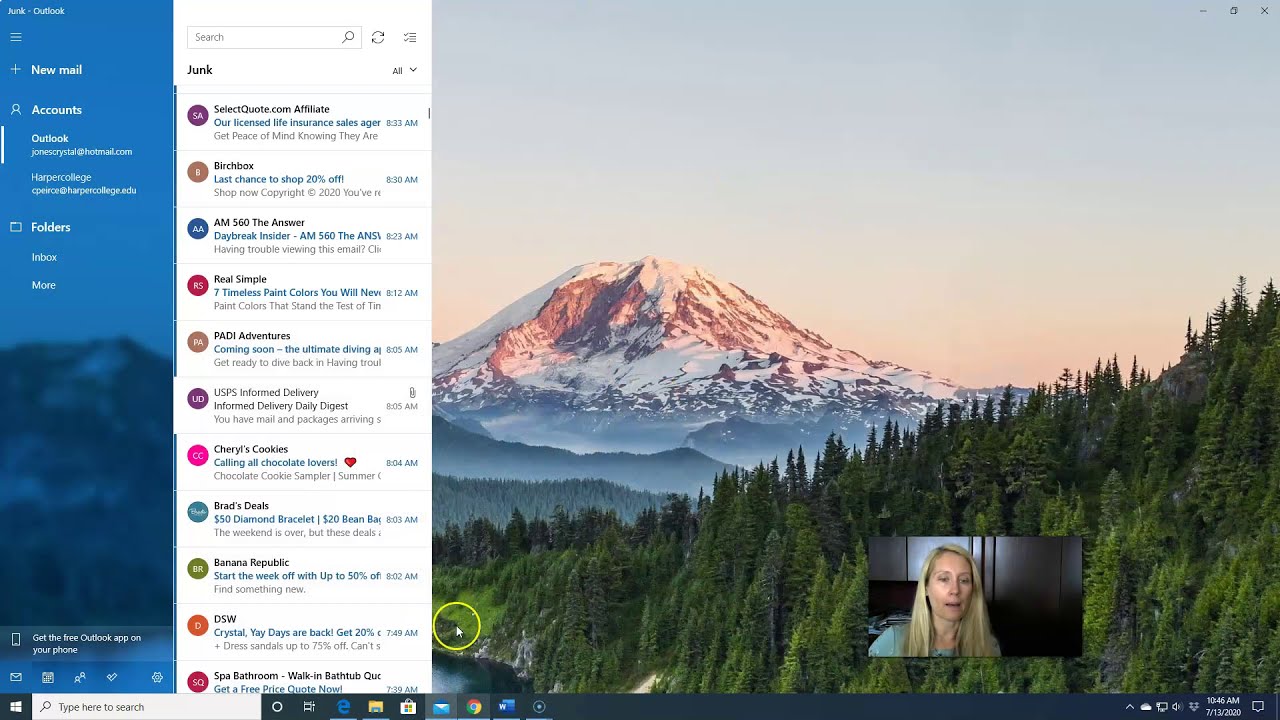The screenshot captures a computer screen displaying a mixture of email interface elements and a scenic screensaver. On the far left, a vertical blue sidebar lists "New Mail," "Accounts," and "Folders," while a white vertical block adjacent to it contains a preview of junk mail messages. The background features a stunning screensaver of a snow-covered, vegetation-free rocky mountain with a bright blue sky. In the forefront of the image, green pine trees cascade down a hillside to a serene lake at the mountain's base. A small circular icon with an arrow is also present within the screensaver. Positioned at the bottom right of the screen is a small video call window showing a blonde Caucasian woman wearing a blue or green top. She appears to be engaged in a conversation, looking down at her screen with her mouth open. This scene likely represents a moment where the user is multitasking with their email and a Zoom meeting, all set against the backdrop of the tranquil mountain landscape.